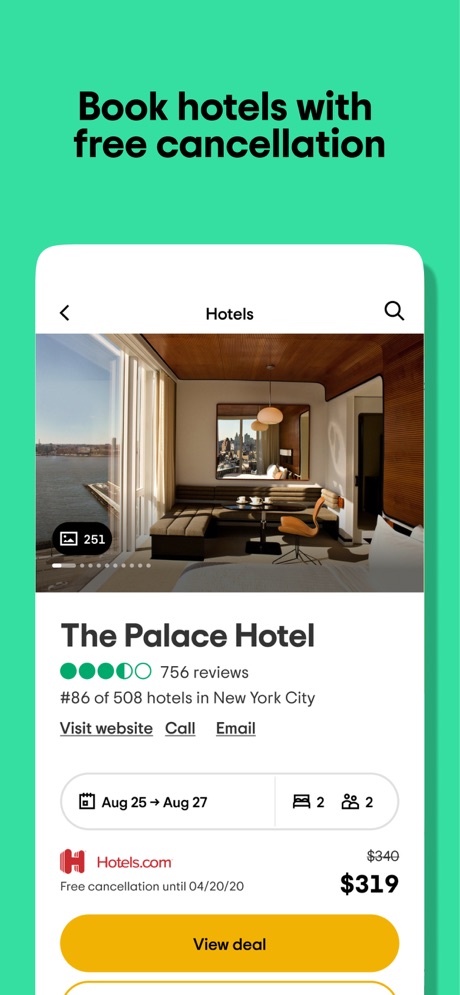The image appears to be an advertisement for a hotel booking service. The background is a light green shade, providing a subtle yet appealing backdrop. The focal point of the advertisement is a large cell phone screenshot occupying the upper section of the image, stretching slightly to the left and right. The cell phone screenshot features a drop shadow on its right-hand side, giving it a three-dimensional, lifted appearance.

Above the cell phone screenshot, in black font, is a two-line text indicating the primary message: "Book hotels with free cancellation." Below this text, the cell phone screenshot specifically showcases details for the Palace Hotel, which boasts a rating of 4.5 stars based on 756 reviews. Additionally, the hotel holds the 86th position out of 508 rated hotels in New York City.